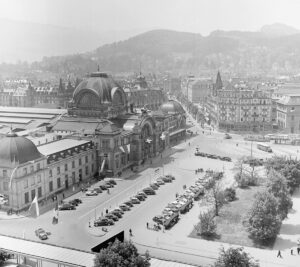This vintage black and white aerial photograph captures a detailed view of a town square from an elevated vantage point, perhaps taken from a tall building or an aircraft. Dominating the left side of the image is a large, ornate building with three distinctive domes, resembling a church or palace. In front of this building is a small parking lot, filled with older-style cars from the 1950s or 60s, parked at an angle, with several people walking around. Adjacent to the parking lot, in the bottom right corner, there is a small grassy area lined with eight or nine trees, some of which are full with leaves while others appear bare. The surrounding cityscape includes multiple blocks with various buildings, and in the far background, the scene is framed by a range of large hills or mountains. The entire composition is richly detailed, capturing a bygone era in monochromatic tones.